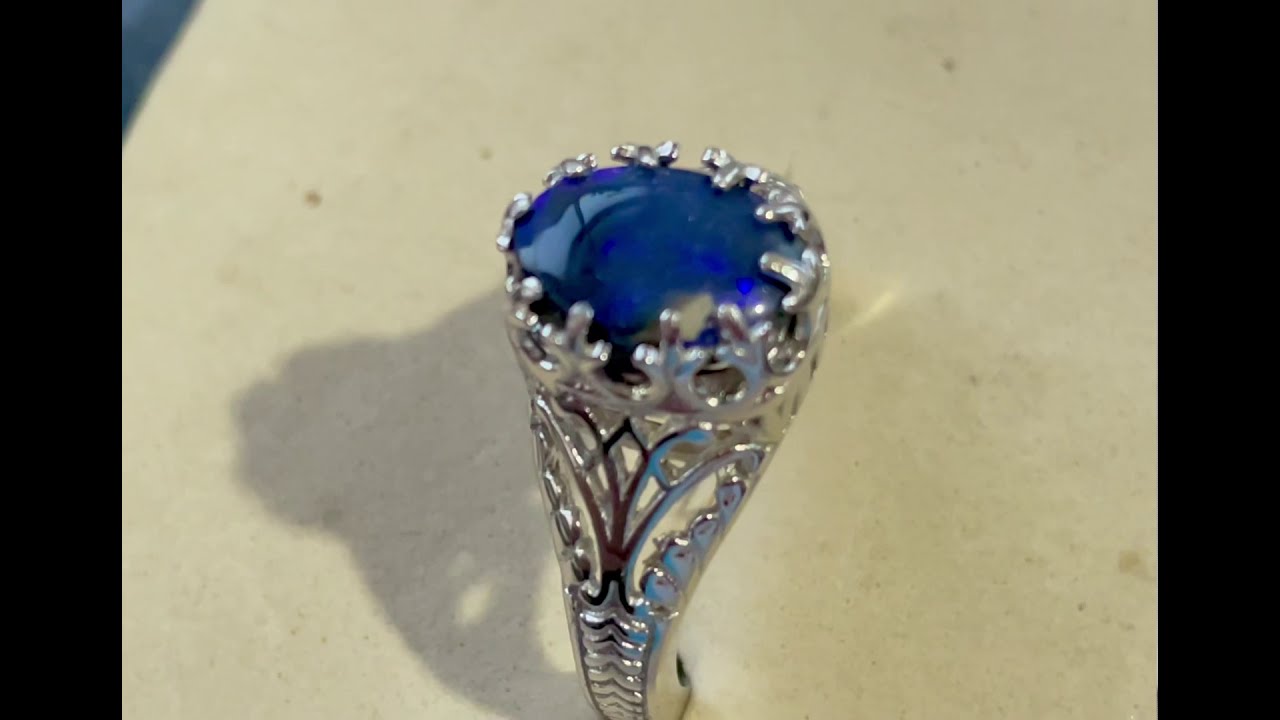The image showcases a carefully detailed picture of a vintage silver ring, prominently featuring a worn blue gemstone that appears to be a dark, possibly synthetic, sapphire. The ring is shown from a top-down angle and stands upright on its own on a slightly blurry white surface speckled with tan accents. The band on the visible side is intricately designed with cutouts, resulting in an ornate, Victorian-style pattern. The ring casts a distinct shadow to the left side on the surface. The gemstone is notably aged, with visible scratches and areas where the color has deteriorated, giving the piece an antique and possibly incomplete look.